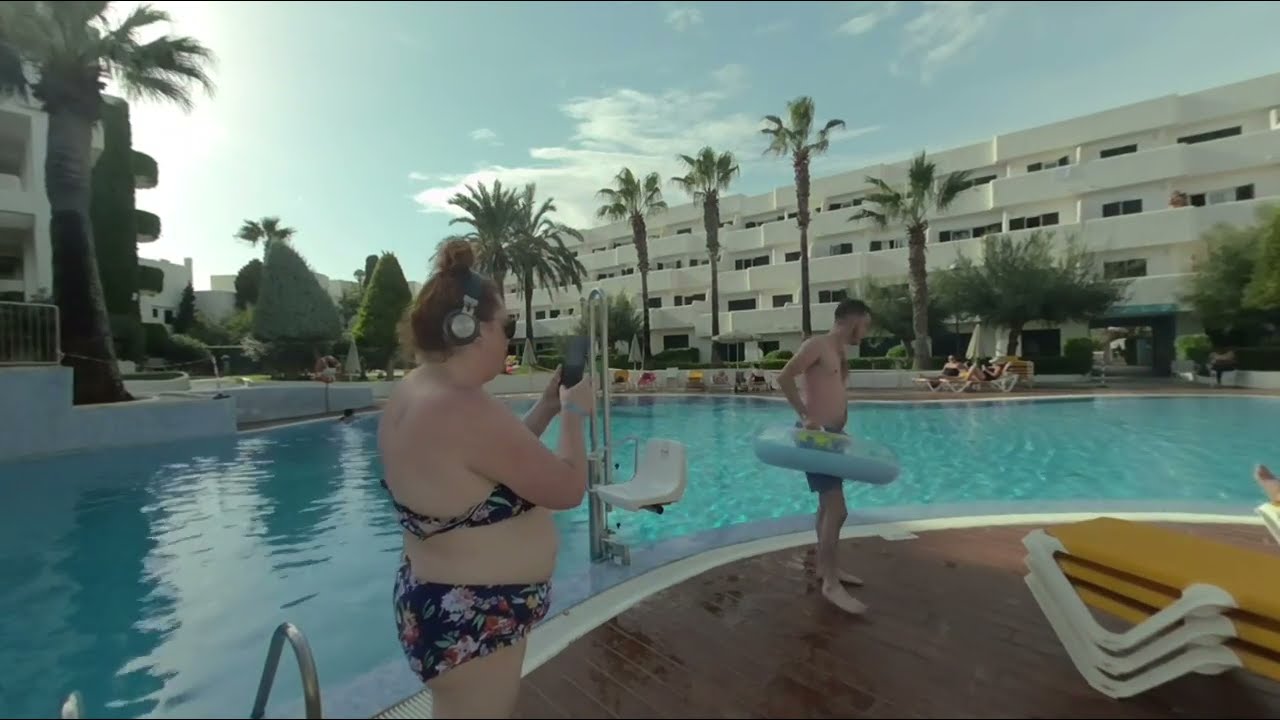This color photograph captures a vibrant poolside scene at a resort or major hotel. In the foreground, a woman with red hair, wearing sunglasses, headphones, and a two-piece bikini, is seen taking a picture with her phone. She stands beside a man who has a blue inflatable inner tube around his waist and is dressed in swimming trunks. Next to them is a stack of empty white chairs, and just behind the woman, pool steps emerging from the clear blue water are visible.

The pool area is surrounded by several palm trees as part of the landscaping, and in the distance, people can be seen lounging in chairs by the pool. The background features a multi-story stone building adorned with balconies and doors, with some individuals standing on the balconies observing the scene below. The image is taken on a sunny day with a few clouds in the sky, adding to the relaxed atmosphere of the resort.